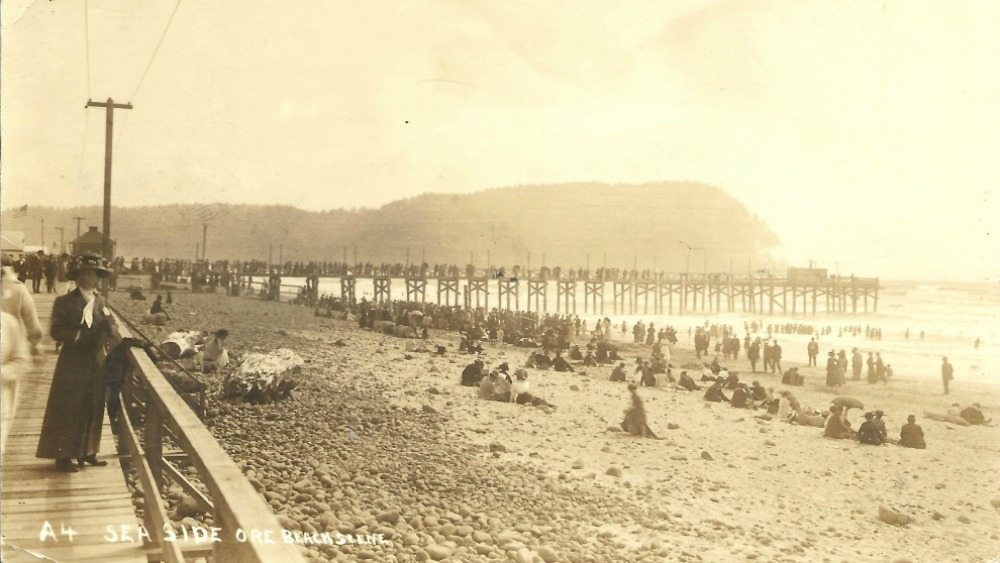This vintage sepia-toned photograph, likely from the early 1900s, captures a bustling beach scene at the Pacific Pier in Seaside, Oregon. The landscape orientation image shows a long wooden pier extending across the center, leading out onto the water. Along the boardwalk on the left, a woman in a long black dress and top hat stands prominently, gazing down toward the rocky beach below where numerous people are scattered. Overhead, a power pole with lines extends upwards, adding to the vintage ambiance of the scene. In the background, a wide hill and some clouds complete the horizon. At the bottom left, handwritten text reads "A4 Seaside ORE Beach Scene," marking the location and era of this nostalgic seaside capture.